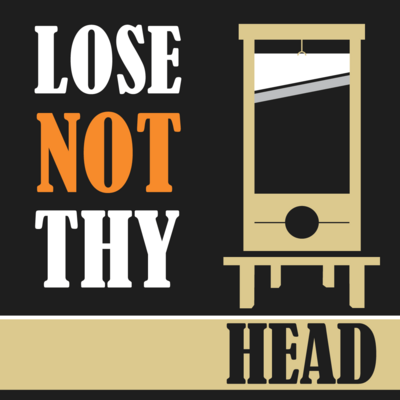The image is a minimalist, cartoony poster featuring the cautionary phrase "Lose not thy head." The text "Lose not thy" is positioned on the left half of the poster, with "Lose thy" in white and "not" in orange. The word "head" is situated at the bottom right, written in black, on a horizontal strip of color that alternates between descriptions of being beige and brown. Above "head," there is an illustrated guillotine with a brown frame and a white and silver blade, raised in the air. The overall background of the poster is primarily black, creating a stark contrast with the text and guillotine. The guillotine and the strip below it match in color. The style is simple and may have been created digitally, making it suitable for use online or as a book cover, as well as a physical poster.